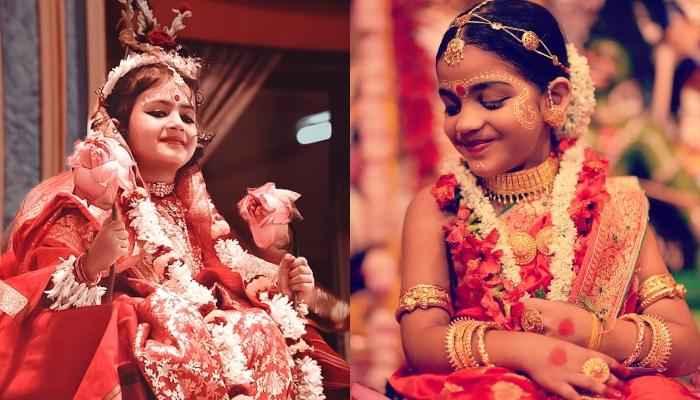This image features two color photographs arranged side-by-side to create a cohesive landscape orientation. Both photographs capture young girls adorned in traditional Hindi attire. They share several similarities including bindis on their foreheads, intricate markings that extend from their brows to their cheeks, and ornate jewelry.

In the left photograph, the girl is seated on an elevated surface, dressed in a long red robe with white fringe down the front, layered over a red and white brocade dress. She wears an elaborate headdress topped with a bird-shaped statue and a decorative feather arrangement. Her neck is adorned with a silver choker necklace and a necklace made of white flowers. She holds two large dried pink roses, one in each hand, and smiles down at the camera, creating an engaging and inviting presence.

The right photograph showcases another girl from head to mid-waist. Her attire includes a sleeveless red dress with golden decorations and a beaded gold collar necklace. She has a gold filigree headdress paired with a head wrap and wears several gold bangle bracelets on her upper arms and wrists. Around her neck, she has two flower necklaces: one made of white flowers and the other of bright red ones. She stands with her hands crossed in front of her, looking down to the left and smiling softly, evoking a serene and elegant mood.

Together, these portraits highlight the cultural richness and beauty of traditional Hindi dress, capturing the young girls' graceful and poised demeanors in a style that can be described as representational realism.